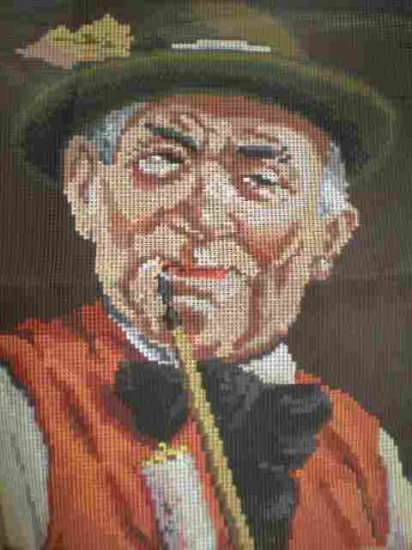The image depicts a meticulously crafted piece of fabric art, resembling a cross-stitch or woven portrait of an elderly Caucasian man. The artwork, which features pixelated details that create a jagged appearance along the edges, showcases muted colors with a predominant brown and olive-green background. The man, with a roundish face, has gray hair on the sides and wears a distinctive hunter green bowler or fedora hat, possibly adorned with a leaf or feather. He sports a white or off-white striped shirt underneath an orange or red vest and is further layered with a black coat. Highlighting his facial features are his prominent, large nose, big ears, and pink lips. Although it's uncertain, he might be holding a pencil-shaped item or a stick with a black, obscure end similar to a pool stick's thickness. With his gaze directed towards his left, at around a 5 o'clock angle, the man also appears to don a voluptuous bow tie. This evocative portrait, likely inspired by early 20th-century designs, conveys a sense of nostalgia and reflects the careful stitching work, evident through the visible stitch marks and intricate texturing.